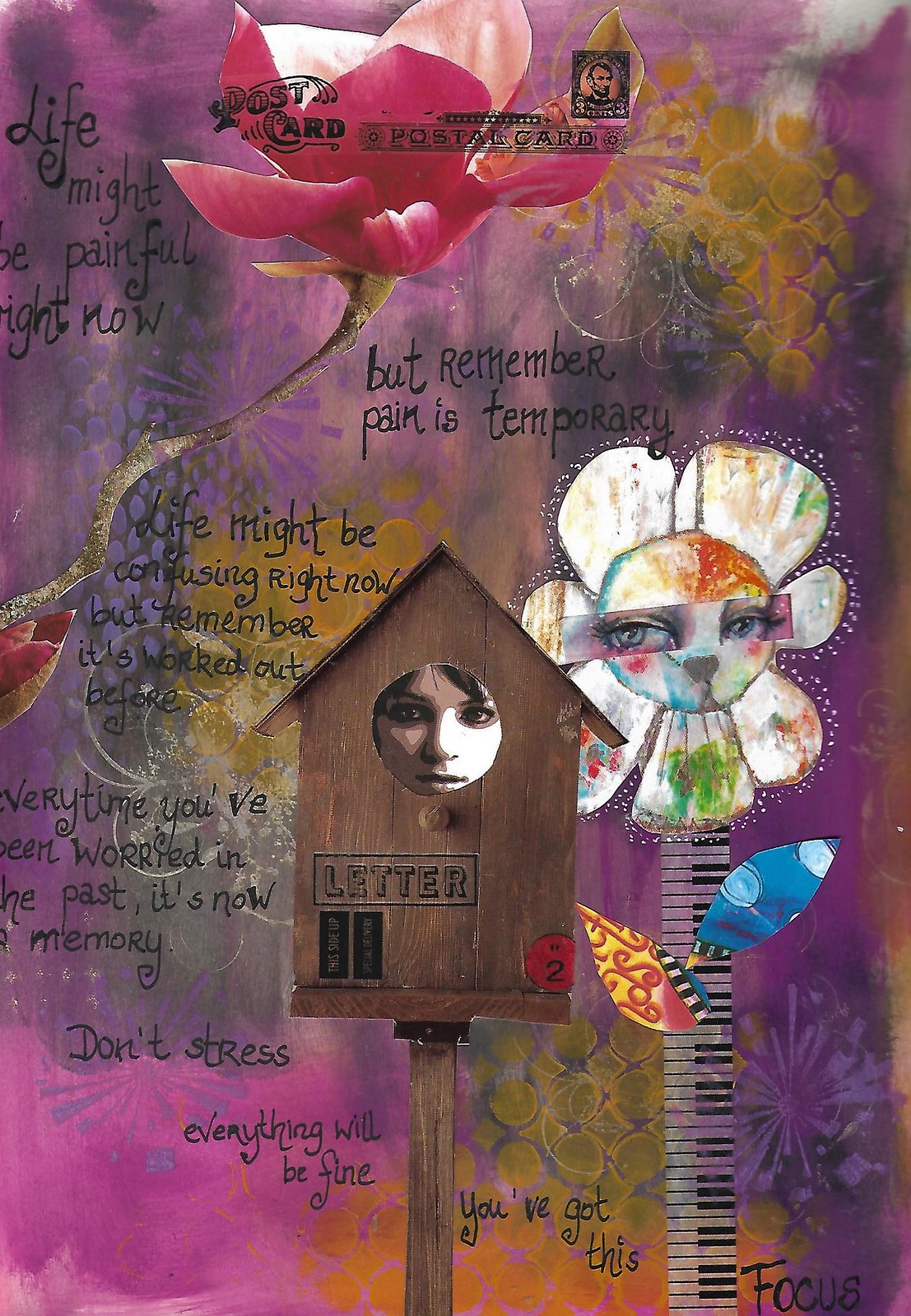The image is a piece of eclectic art featuring a rich, purplish-pink background that captures the eye immediately. At the center of the composition stands a birdhouse with a distinctive twist: inside its window is a black-and-white portrait of a person's face, lending an enigmatic touch. On the birdhouse, the word "LETTER" is stamped prominently, and the number "2" is delicately positioned at the bottom right corner.

To the right of the birdhouse, there is a creatively designed element that resembles piano keys intertwined with a flower stem, leading to a white flower adorned with green and red hues. Intriguingly, the center of the flower holds the eyes of an unknown animal, adding a curious focal point.

At the top of the artwork, a red flower is illustrated, and nestled within one of its leaves is the word "POSTCARD." Scattered across the card is an uplifting message that reads: "Life might be painful right now, but remember, pain is temporary. Life might be confusing right now, but remember, it worked out before." This message continues towards the bottom, encouraging the viewer with, "Stress everything will be fine. You've got this," and culminating with the word "FOCUS" in the lower right corner.

This imaginative and layered artwork blends elements of surrealism with motivational inscriptions, creating a captivating and thought-provoking piece.